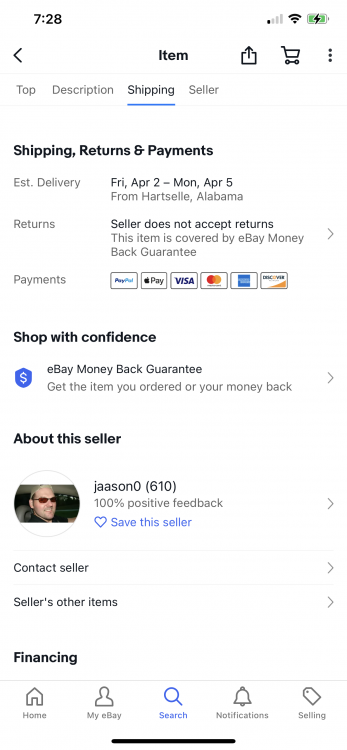A mobile phone screen displaying an eBay transaction is shown in the image. The purchase amount is $7.28. The phone's status icons indicate one bar of signal strength, Wi-Fi enabled, and a fully charged battery with an active charge denoted by a green bar and a lightning bolt icon.

At the top of the screen, navigation symbols include a left-pointing arrow and a less-than sign, suggesting a way to go back. Further icons represent "item" (depicted by a piece of paper with an arrow), a shopping cart, and a menu symbolized by three vertical dots.

A faint gray horizontal line separates the sections of the menu, showing tabs for "top," "description," "shipping," and "seller." The "shipping" tab is currently selected, highlighted by a blue line underneath it.

In the shipping section, details include "shipping returns and payment" with an estimated delivery date from Friday, April 2nd to Monday, April 5th, shipping from Hartsell, Alabama. Returns are not accepted by the seller, but the item is covered under the eBay Money-Back Guarantee. 

Payment options accepted are PayPal, Apple Pay, Visa, MasterCard, American Express, and Discover, each illustrated by their respective icons. A "Shop with confidence" section reassures buyers with a dollar sign inside a shield, stating "Get the item you ordered or your money back." 

The seller section presents an image of a man with sunglasses, blonde hair, and stubble, labeled "JAASON0," with a feedback score of 610, all 100% positive. A blue heart icon and the text "Save the seller" are present, as well as an option to contact the seller.

Additional options include "Seller's other items," "Financing," and a bottom menu with icons and labels for "Home," "My eBay," "Search" (highlighted in blue), "Notifications," and "Selling." Each option is represented by relevant icons such as a house, person, magnifying glass, bell, and price tag respectively.